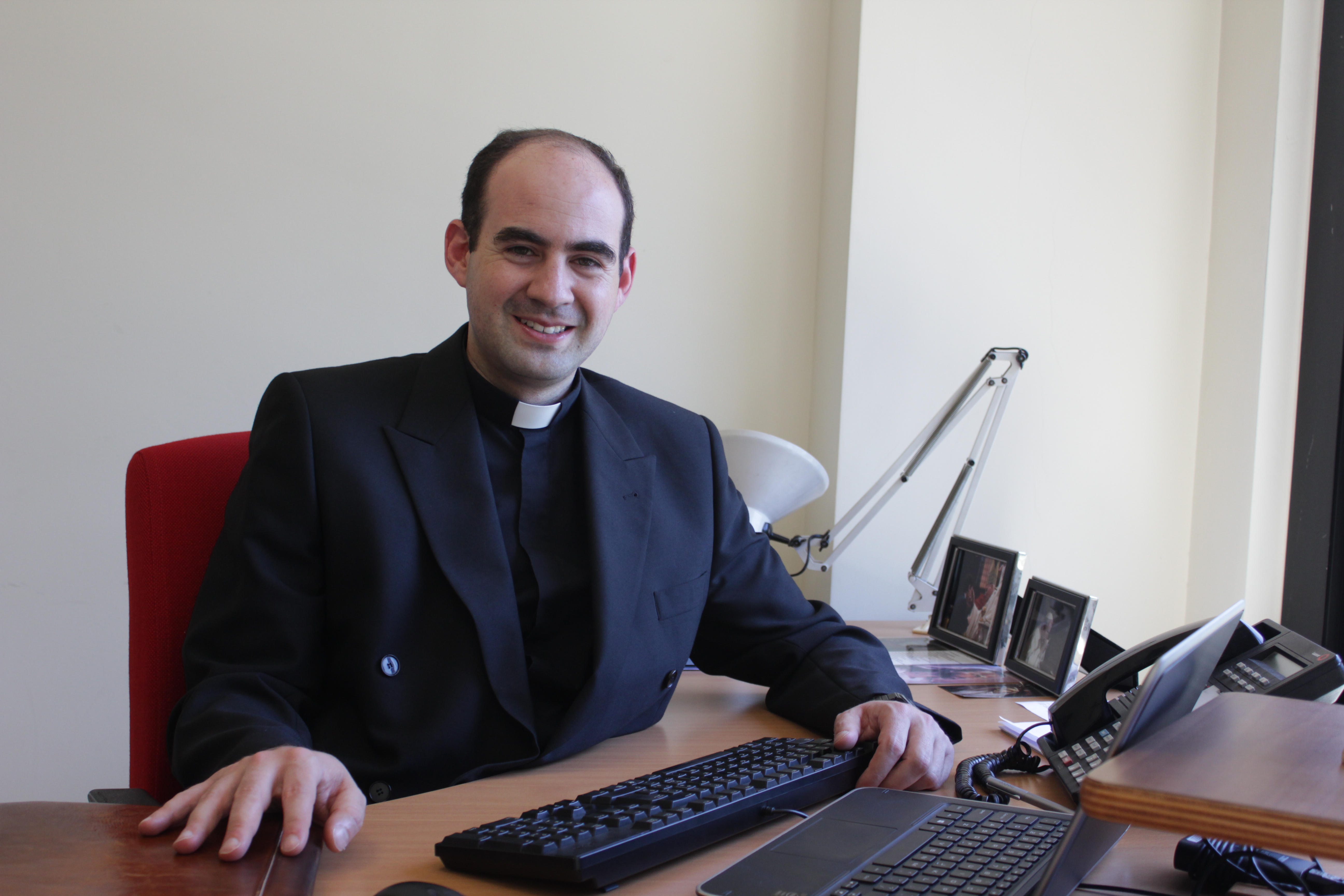This photograph captures a balding white man with very thick eyebrows seated at a wide, circular computer desk that centers around him. He is dressed in a black tuxedo jacket with a black dress shirt collar, suggesting a possible religious figure, such as a priest, given the formal attire and choker-like collar. The man, who is smiling, is seated in a red chair and positioned facing the camera.

In front of him on the desk is a light brown laptop with blue accents and a black keyboard, indicating it is a Windows computer. To his right, a black landline phone is situated. The desk also holds two framed photographs and features a retractable desk lamp folded over in the background. The absence of text or wording, along with the array of off-white, tan, and brown tones, suggests the setting is indoors, likely in his office, with daylight filtering through a window on the right, casting light on the wall. The man’s hands are placed in front of him on the desk and keyboard, capturing a focused yet approachable moment in his personal workspace.